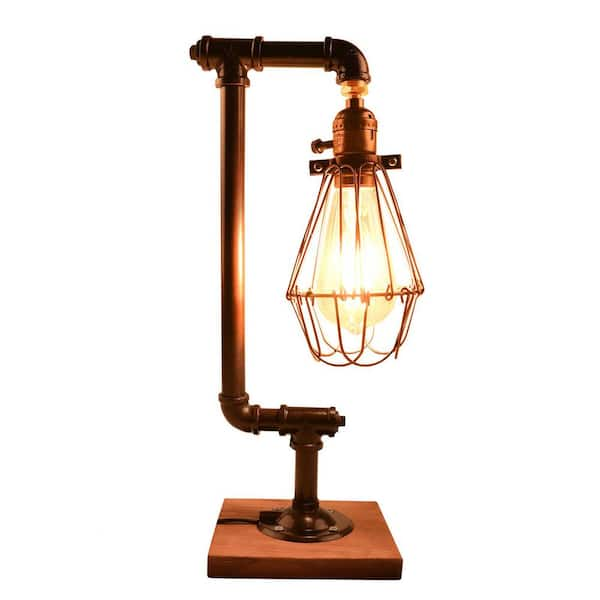The photograph features a uniquely designed lamp that resembles a lantern, set against a white background. The lamp sits on a square wooden base, approximately a four-by-four inch in size, which supports a network of metal pipes forming elbow joints. These pipes, along with the rest of the metal components, exhibit a bronze or copper color. The piping structure supports a dangling light bulb, enclosed within a wire cage that mirrors the bulb's shape. The cage and bulb emit a bright white light at the center, surrounded by a softer amber and yellow glow, creating a visually appealing contrast. The overall construction includes a combination of steel and copper-colored elements, lending an industrial and vintage aesthetic to the lamp.